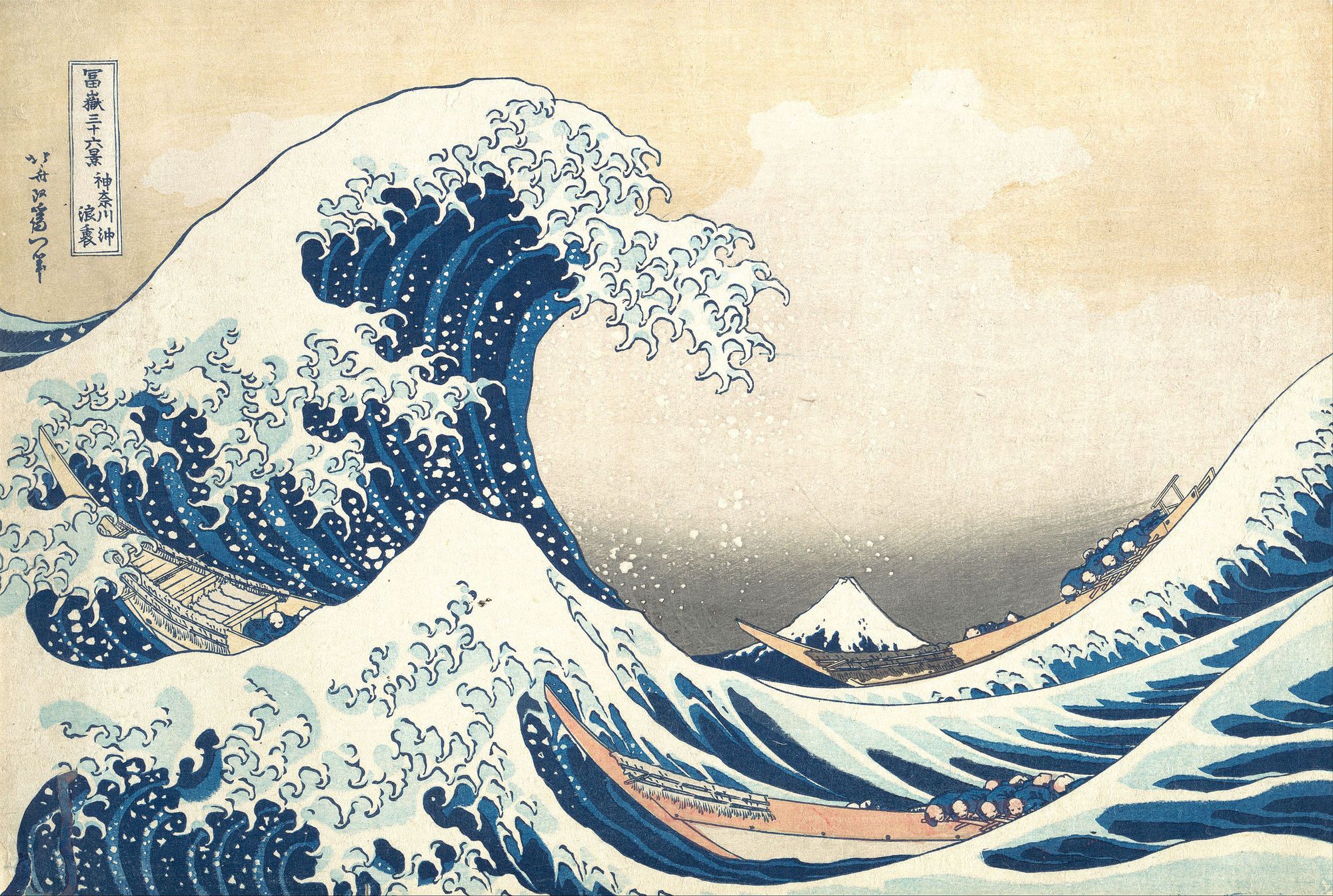The image portrays a dramatic and stylized scene of a large, violent wave, often recognized from famous Japanese art. The dark blue wave, with dynamic white foam indicating its tumultuous nature, appears ready to engulf three long, pointed boats. The boats, brown in color, are occupied by people dressed in blue uniforms who are crouching in fear, evidently frightened by the impending force of the sea. Surrounding the chaos, the sky is a light beige with scattered clouds, creating a stark contrast with the powerful waves below. On the upper left side of the image, there is text written in an Asian language, adding to the cultural and historical depth of the scene, reminiscent of tales like the Japanese kamikaze or "divine wind."